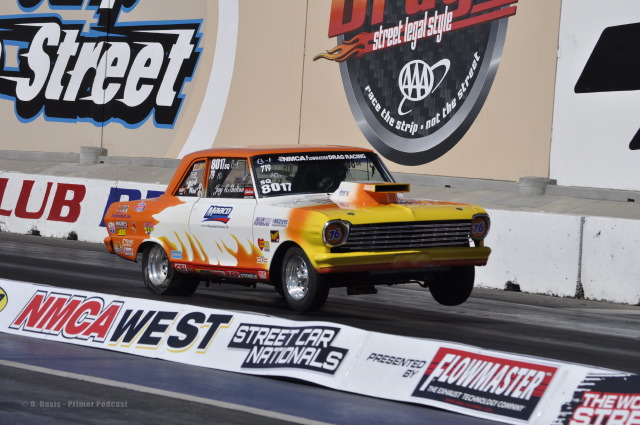This photo captures a dynamic moment at a street race track. A vintage race car, distinguished by its boxy design and vibrant paint scheme, is depicted in the heat of action. The car features a striking combination of orange and white colors with yellow on the bumper and front part of the hood, transitioning into flames along the sides. It prominently displays the number 76 on its headlights and the number 8017 on the windshield. Logos of various sponsors, such as NMCA and Flowmaster, adorn the car, including on the windshield and glass windows.

The vehicle is shown mid-race, with at least two of its tires lifted off the ground, suggesting rapid acceleration or a powerful launch from the start line. In the background, graffiti art on the track walls features slogans like "Race the strip, not the street" and logos stating "Street Car Nationals presented by Flowmaster." The scene is framed by barricades covered in sponsor logos, and a watermark by D. Davis Primer Podcast is visible in the bottom left corner. The image captures the essence of high-speed racing amidst a blend of artistic urban backdrop and commercial branding.